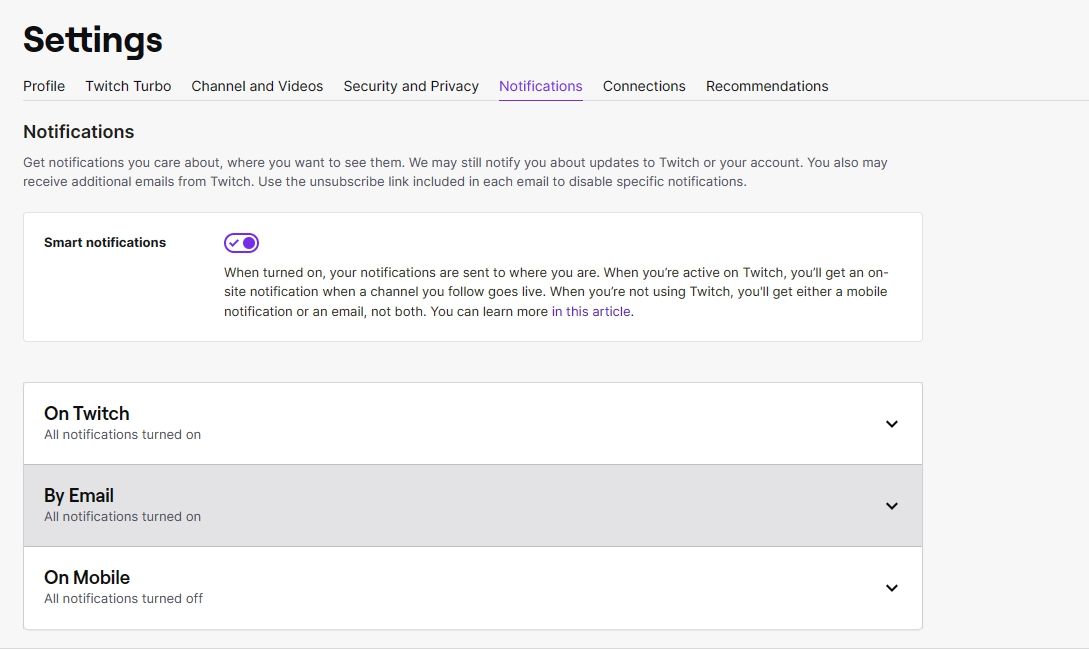The image appears to be a screenshot of Twitch's settings page, specifically focused on the notification settings. At the top left corner, there is a prominent "Settings" label in black. Directly below that, a horizontal menu lists various sections in the following order: Profile, Twitch Turbo, Channel and Videos, Security and Privacy, Notifications, Connections, and Recommendations. Among these, the "Notifications" tab is highlighted in purple, with a purple line underneath it.

The main section begins with a header stating "Notifications." Below this header is a subheader that reads, "Get notifications you care about where you want to see them. We may still notify you about updates to Twitch on your account. You also may receive additional emails from Twitch. Use the unsubscribe link included in each email to disable specific notifications."

A prominent feature in this section is the "Smart Notifications" option, presented in a white rectangle. This option is represented by a toggle switch with a purple outline, a purple tick on the left, and a purple circle on the right, indicating that it is currently turned on. The accompanying text explains that with Smart Notifications enabled, notifications are sent based on your activity: on-site notifications appear when you are active on Twitch, while mobile notifications or emails are sent when you are not using Twitch. A hyperlink, labeled "learn more in this article," provides additional information.

Below the Smart Notifications section are three more rectangles:

1. **On Twitch** - This section, set against a white background, indicates that all notifications are turned on.
2. **By Email** - Featuring a gray background, this section also shows that all notifications are turned on.
3. **On Mobile** - Another section with a white background, it indicates that all notifications are turned off.

Each of these sections features a downward-pointing arrow on the far right, indicating they are drop-down menus for further customization. There is no additional text in the image.